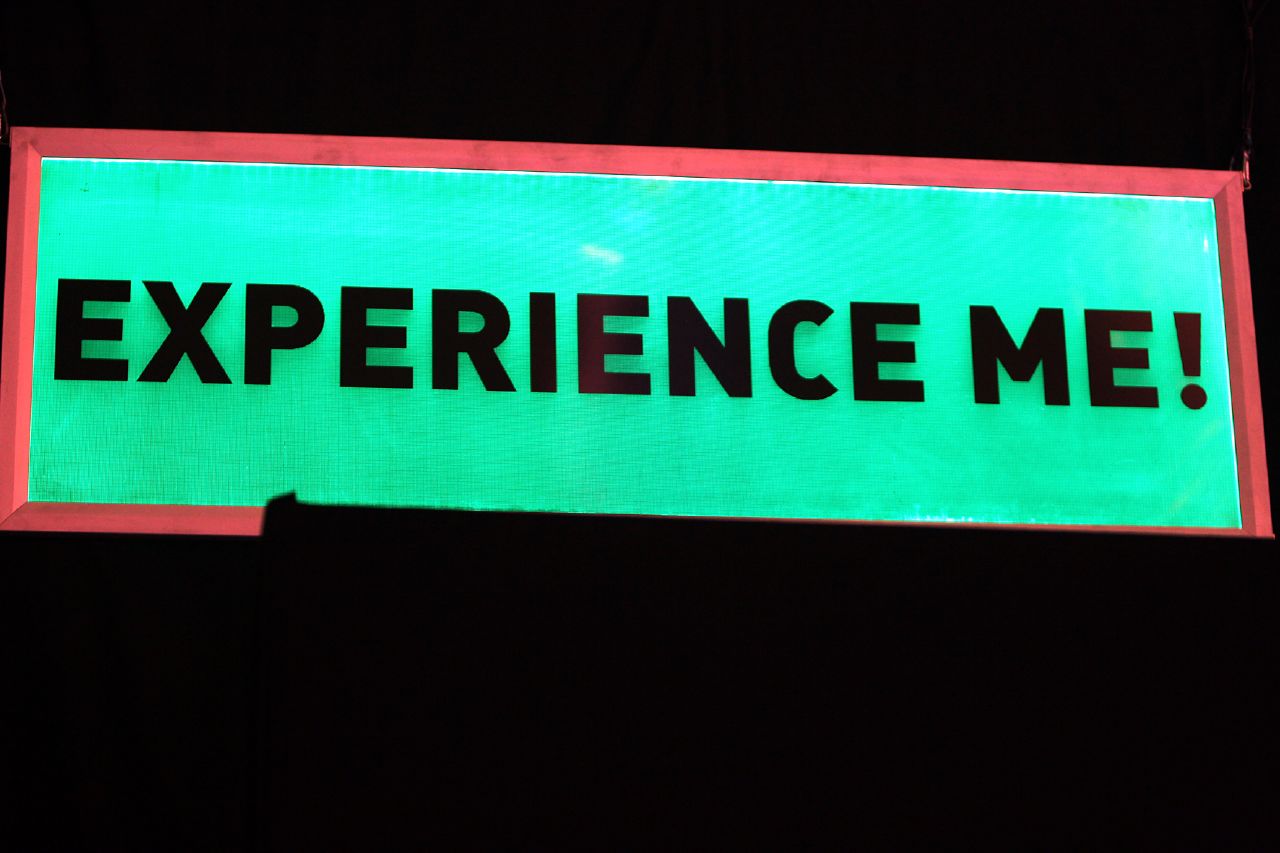The image depicts a digital neon sign with a vibrant turquoise background and bold, capitalized black letters that spell out "EXPERIENCE ME!" The sign has a rectangular shape and stretches prominently across the dark, predominantly black background, making it the focal point. Surrounding the turquoise area is a pinkish-red wooden-looking frame that adds a colorful contrast. However, the bottom right portion of the sign's border is obscured by a shadow, slightly cutting off the frame. The vivid colors and sharp text create a striking visual against the empty, pitch-black backdrop.